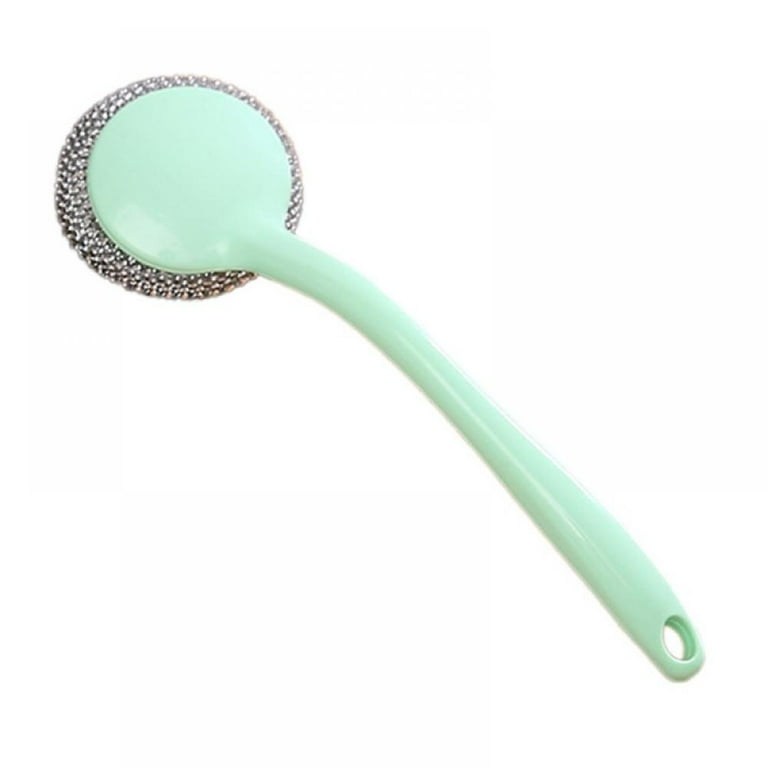The image showcases a dish scrubber featuring a light mint green, seafoam-colored plastic handle with a hole at the bottom right corner for hanging on a hook. The handle is smoothly connected to a circular end, which houses a shiny, uniform metal mesh resembling a more structured version of a Brillo pad. The metal scrubbing surface is positioned at the top left of the image. The entire product appears new and clean, presented against a stark white background without any additional text or packaging.